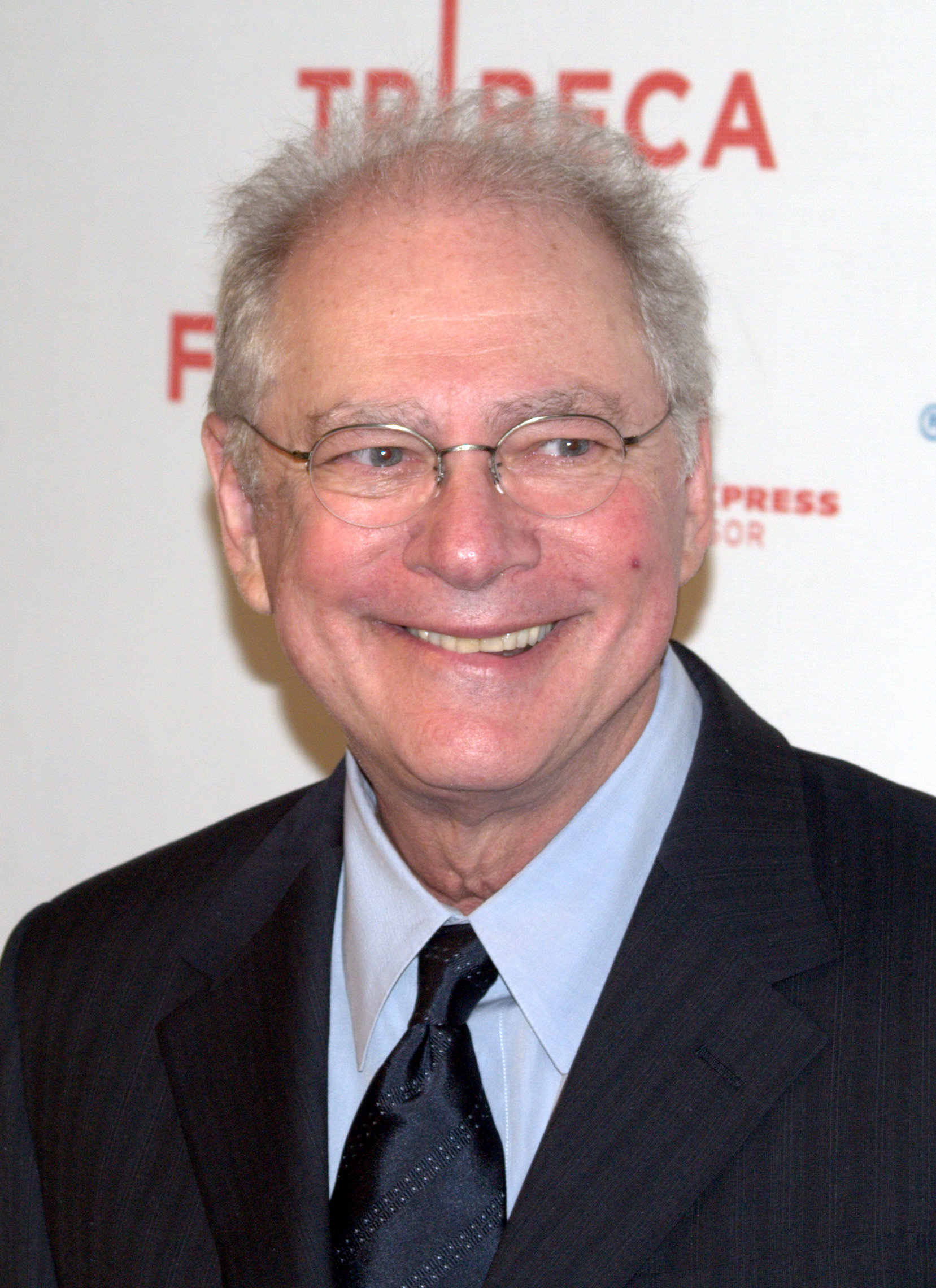In the photo, an elderly white male with sparse, short gray hair, light-colored eyes, and thin-rimmed eyeglasses is smiling warmly while looking slightly to the right. He is dressed in a dark gray or black pinstriped suit, complemented by a white undershirt and a black satin tie adorned with white dotted stripes. The man stands against a white wall featuring red printed words, including "Tribeca" and "press," which are partially obscured by his head. The setting appears to be indoors, possibly at a film festival event, and the composition centers him prominently in the image.